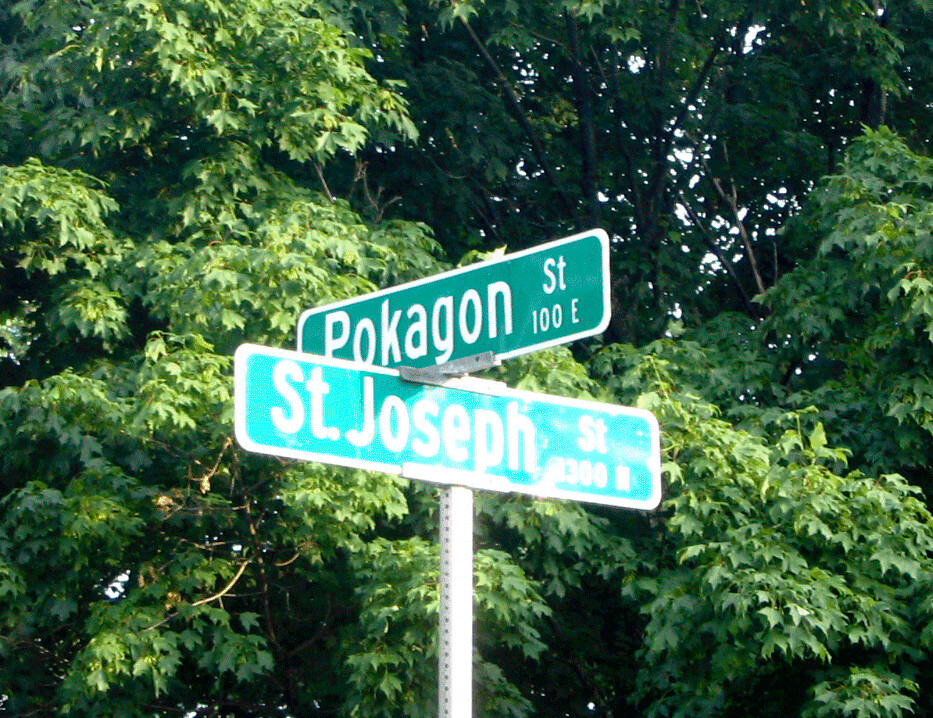This image captures an intersection where two street signs meet. The top sign reads "Pocahontas Street, 100 East," while the intersecting sign below, albeit slightly blurry, appears to read "St. Joseph Street, 300 North." Both signs are affixed to a sturdy metal pole, likely embedded in the sidewalk for stability. In the backdrop, a dense cluster of tall trees, lush with fully bloomed green leaves, frames the scene. Through the gaps between the foliage, one can discern that it is a bright and sunny day. The street names are prominently displayed in white lettering against the green background of the signs.